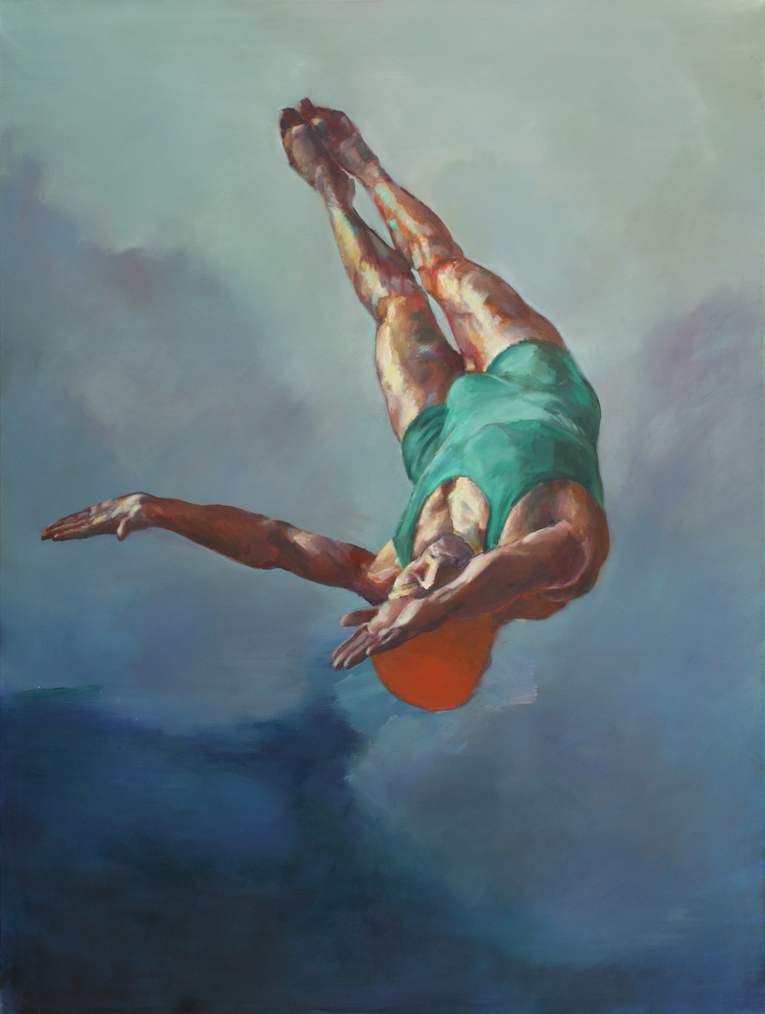This painting, titled **"Fluge (German Fragments)"** by **Daniel Sambo-Richter**, is a color oil painting in a portrait orientation. It depicts a high diver, likely a male, captured in mid-air during an impressive dive. The diver is viewed from below, making his feet and legs appear overhead, his body twisted slightly to the left, with his head pointed downward toward a dark blue body of water. 

He is attired in a green one-piece swimsuit that extends over his shoulders like a tank top. An orange rubber diving cap rests snugly on his head. The diver's arms are extended above his head, palms facing up, with his legs perfectly straight and feet together, suggesting a well-executed dive. 

The background features a cloudy sky, with variations of white, gray, and dark gray clouds, blending into a gradient of light to dark blue as it reaches the horizon. The diver's skin tones, suggestive of a Caucasian man with tanned legs and arms, add a realistic touch to the painting. The style can be described as contemporary realism, focusing on figurative elements that bring the scene to life.